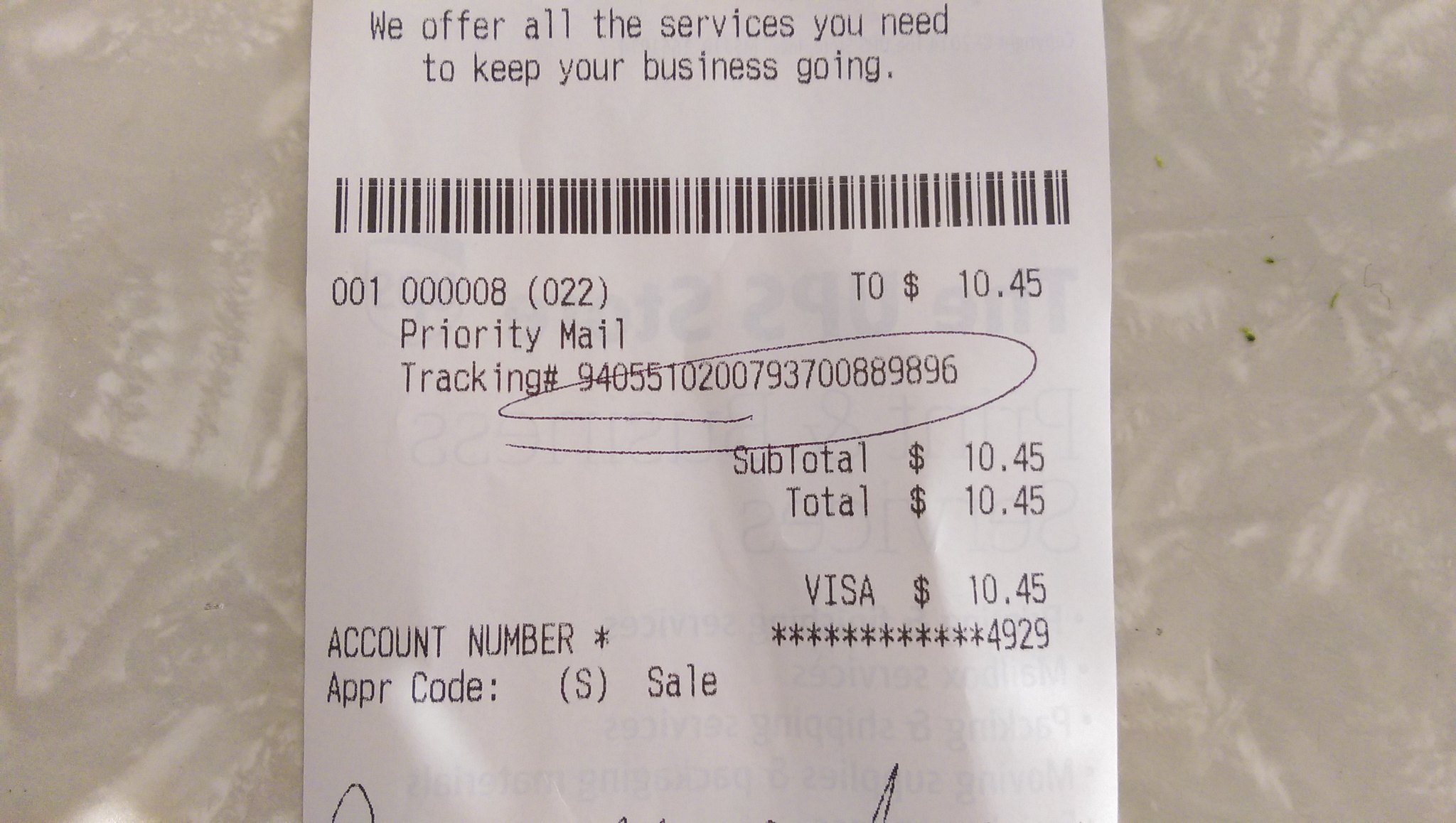This detailed close-up image showcases a USPS receipt prominently positioned against what appears to be a white and beige marble countertop. The background on either side of the receipt features a gray and white pattern, adding a contrasting frame to the document. The receipt itself is printed in black ink and starts with the sentence: "We offer all the services you need to keep your business going." Directly below this statement is a partially visible barcode followed by a series of numbers: "001 00008 (022) Priority Mail." The receipt also features a long tracking number, "9405510200973700889896," which is circled in pen. The financial details indicate a total cost of "$10.45," which is consistently listed as the subtotal, total, and the amount charged to a Visa card. The receipt displays the last four digits of the account number as "4929" and includes an APPR code. The document appears to have been signed, marking the transaction as complete. This comprehensive receipt captures the essential details of a USPS transaction for sending a package.